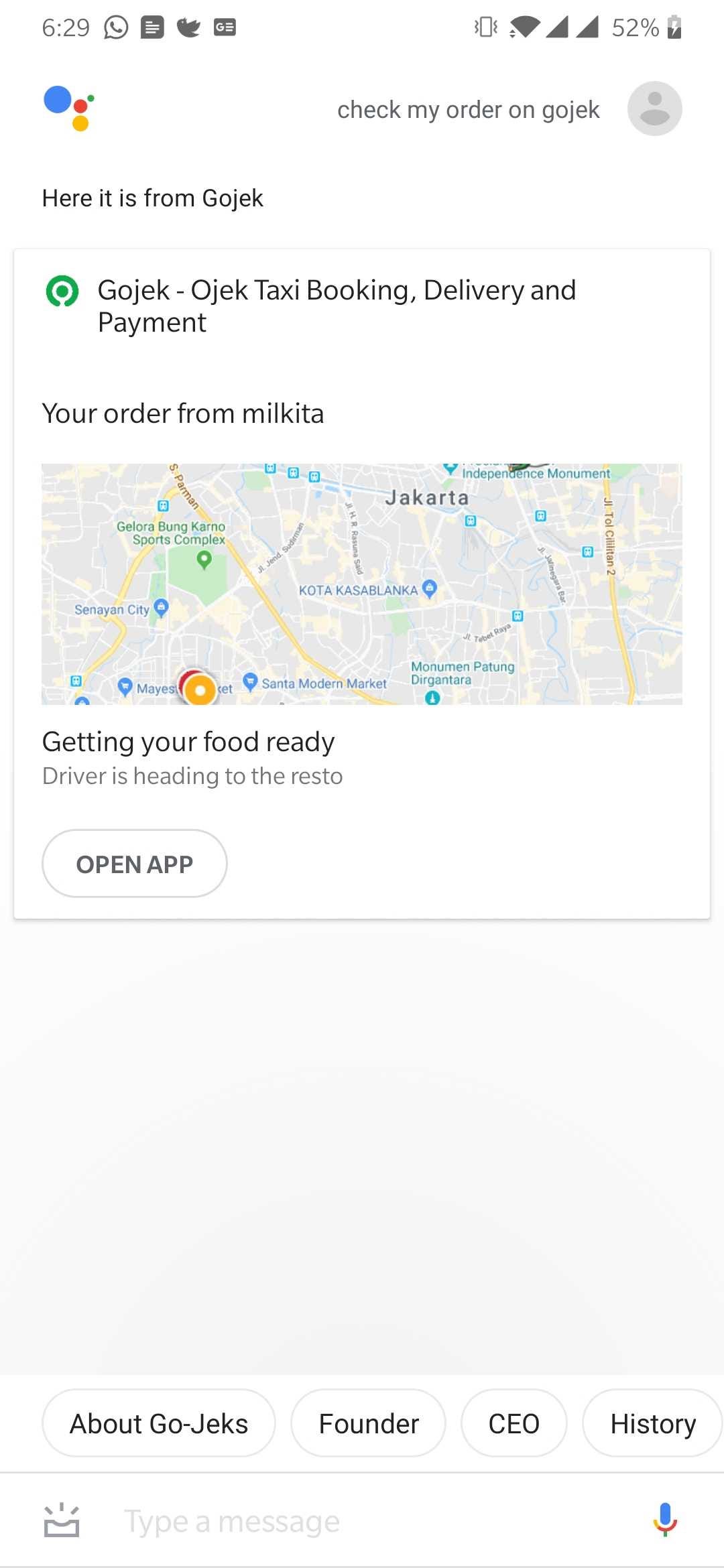Screenshot of a Mobile Device's Webpage: A Detailed Account

In this photographic image, a screenshot captures a webpage viewed on a mobile device. The top status bar reveals it was taken at 6:29, with Wi-Fi enabled, a strong carrier signal, and battery life at 52%. Social media icons for Twitter and WhatsApp are also visible at the top.

The main content of the screenshot focuses on a service from GoJek, as highlighted by the presence of various colored circles—blue, green, red, and yellow—likely part of GoJek's branding. Prominently centered is the text "Check my order for GoCheck" accompanied by a gray profile button. Further down, it says "Here it is from GoJek," indicating the service being used.

Additionally, a green circle with a white border contains the text "GoJek," pertaining to their suite of services including OJek (motorcycle taxi), taxi booking, delivery, and payments. An order from Milkita is mentioned, with a map of Jakarta displayed in shades of gray, yellow, green, and blue indicating the location.

Notably, the map states "Getting your food ready. Driver is heading to the resto," followed by a prompt to "Open app." Towards the bottom part of the screenshot, information about GoJek’s founder, CEO, and company history is briefly visible. 

Complementing the overall interface theme, a Google microphone icon, displaying its recognizable blue, red, yellow, and green colors, is also visible.